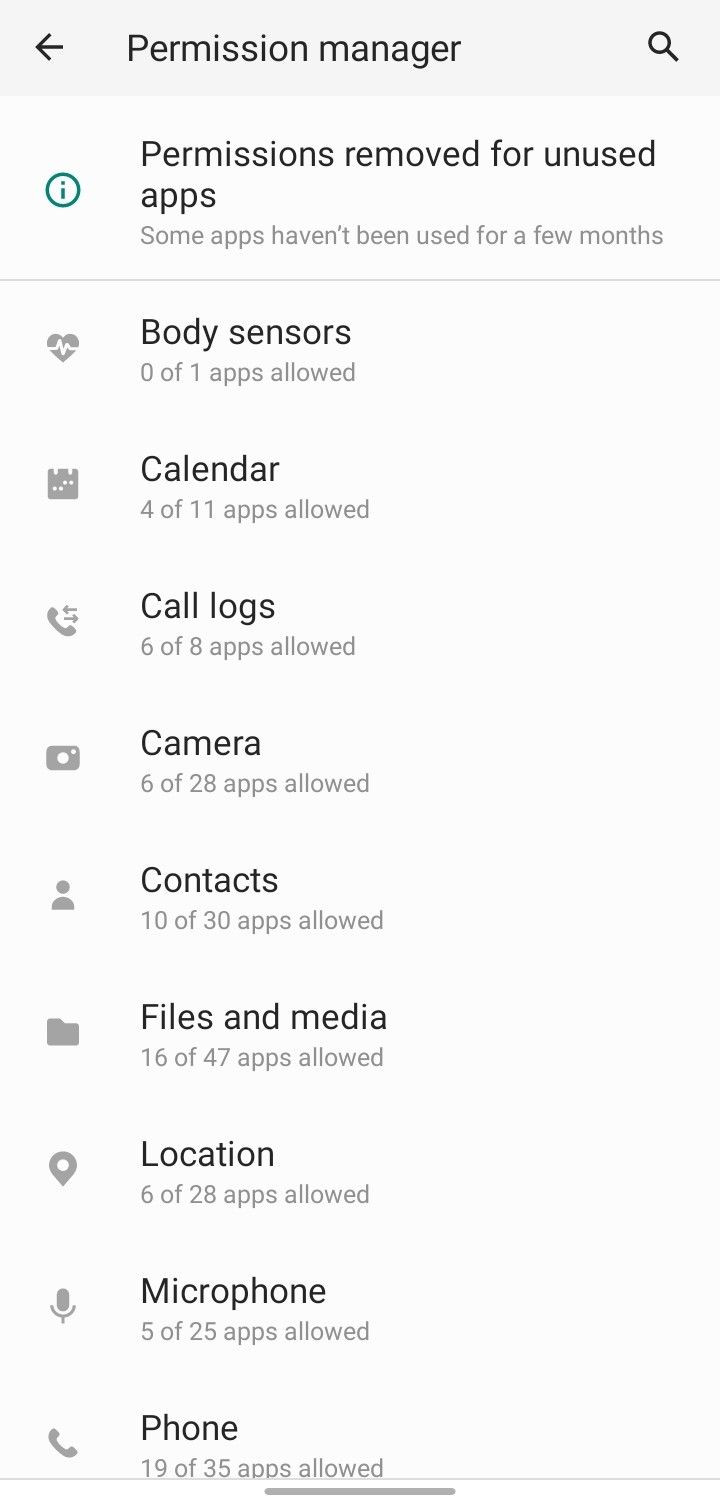This is a detailed screenshot of the Permission Manager app taken on a smartphone. At the top, there's a search bar labeled "Permission Manager," flanked by a left-facing arrow on the left and a magnifying glass icon on the right. Beneath the search bar, a section titled "Permissions removed for unused apps" is highlighted with a green eye icon and a circular "info" icon, providing additional information about this feature. 

The text explains, "Some apps haven't been used for a few months," followed by a categorized list detailing the number of apps permitted for specific permissions out of the total apps available:

- Body Sensors: 0 of 1 apps allowed
- Calendar: 4 of 11 apps allowed
- Call Logs: 6 of 8 apps allowed
- Camera: 6 of 28 apps allowed
- Contacts: 10 of 30 apps allowed
- Files and Media: 16 of 47 apps allowed
- Location: 6 of 28 apps allowed
- Microphone: 5 of 25 apps allowed
- Phone: 19 of 35 apps allowed

The background of the screenshot is white, with most of the primary text rendered in black and the secondary text, denoting the apps allowed, in gray.